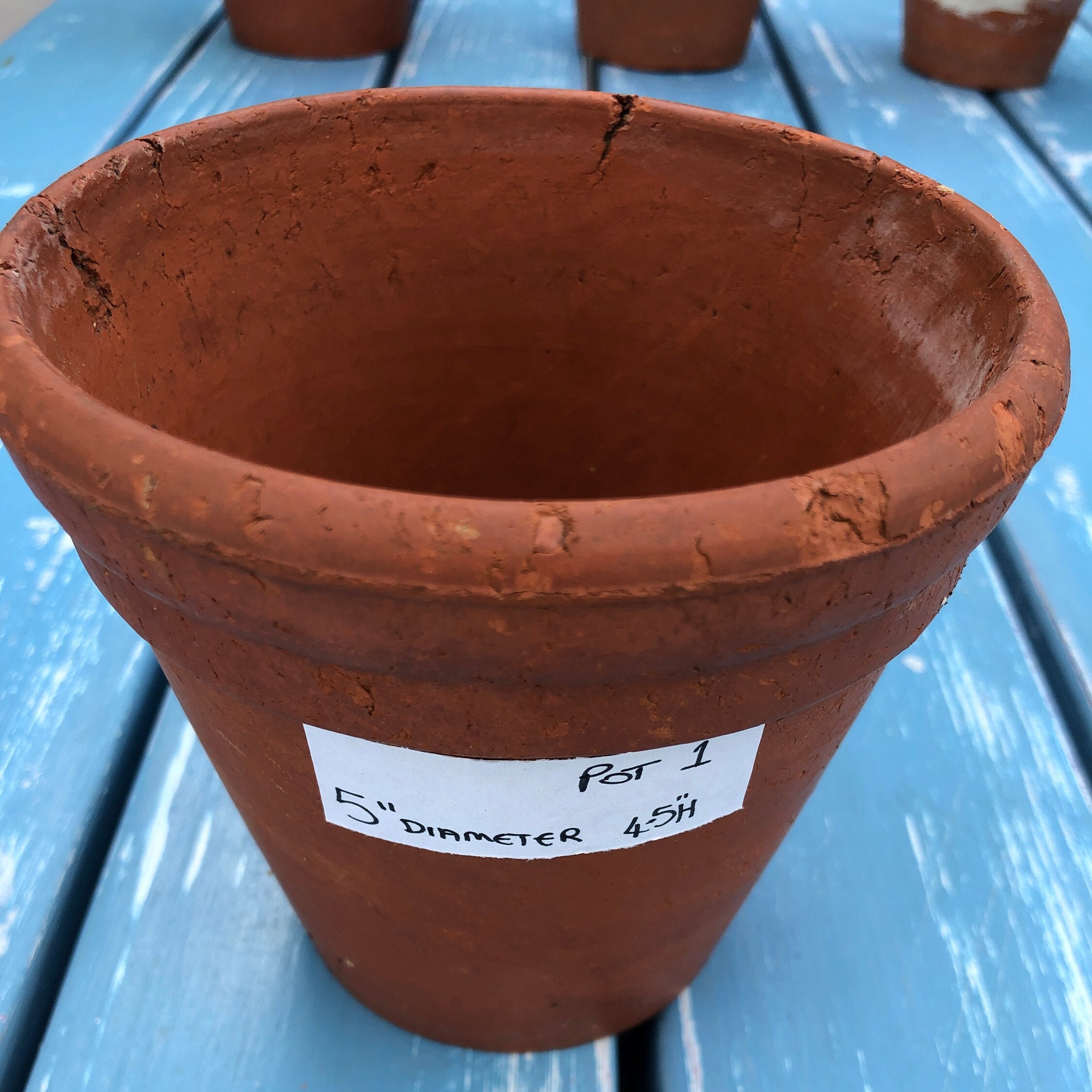This is a detailed photograph of a rust-colored clay planter pot situated outdoors. The pot has a visibly cylindrical shape at the top that narrows towards the base. It features several chips and cracks, common in ceramic vessels. A white label on the front of the pot reads "Pot 1," "5 inch diameter," and "4 to 5 H," written in black marker. The pot is placed on a blue-painted wooden surface with noticeable white streaks and large separations between the planks. In the background, there are three more similar clay pots, visible only by their bases. The lighting in the image suggests it was taken outdoors. The pot's texture transitions from smooth to rough in certain areas, highlighting its rustic charm.